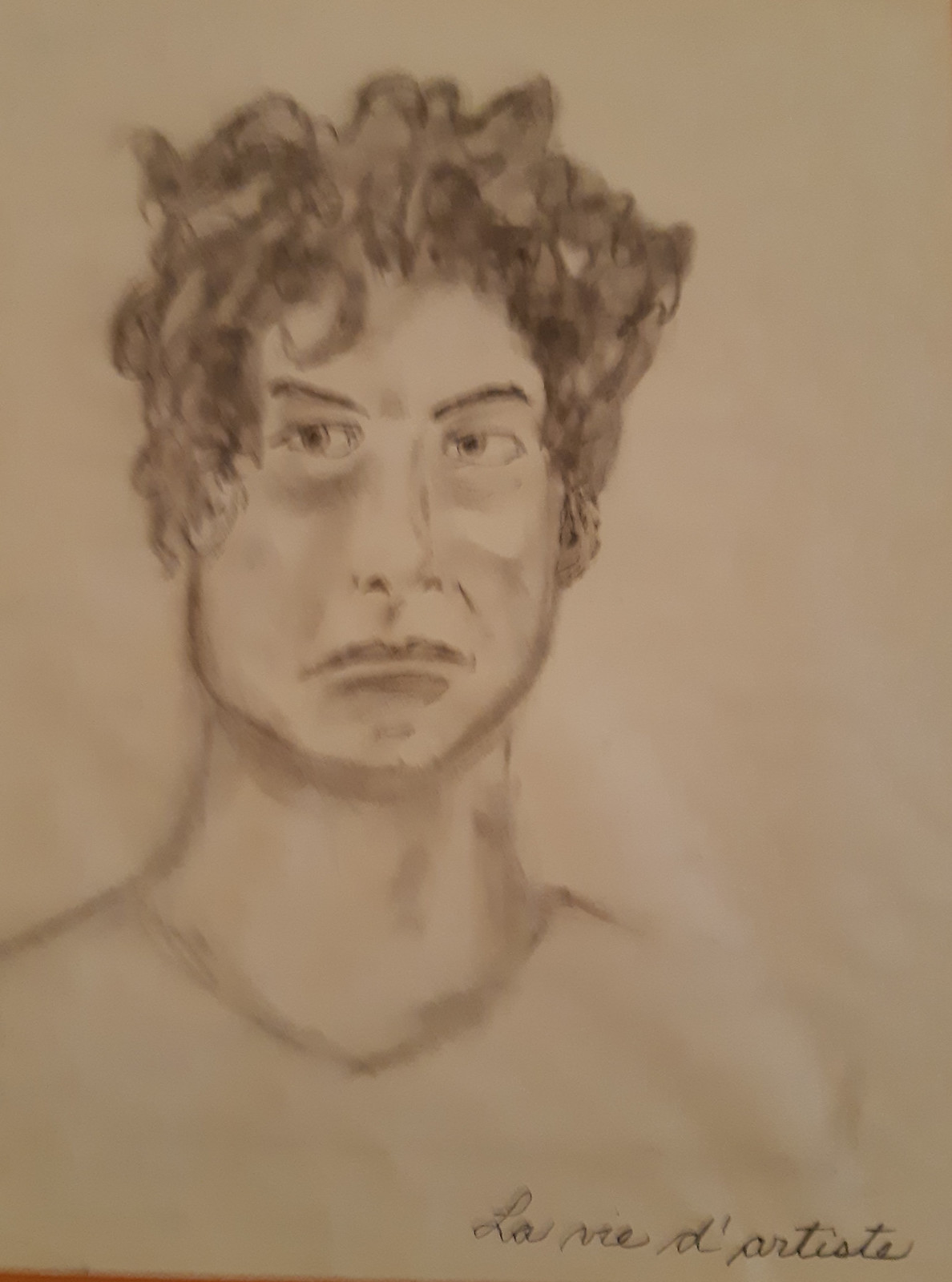This is a detailed black-and-white sketch, likely done in pencil or charcoal, of a man’s face, neck, and upper torso. It appears on a cream-colored piece of sketch paper and has a signature in French at the bottom right corner, reading "La Mare de Artista" or "La Mer de Baptiste," likely the artist's signature. The man in the portrait has a full head of slightly disheveled brown hair and distinctive, upward-curving eyebrows. His facial features include eyes that are a bit offset, a long nose bridge, and a frowning mouth that highlights his rounded lower chin. His strong neck and broad shoulders suggest a muscular build. The shading and highlights give depth to his face, making it seem very illustrative. He seems to be wearing a t-shirt, although some details are not as clear. Overall, the portrait captures a solemn expression with intricate attention to facial features and hair texture.